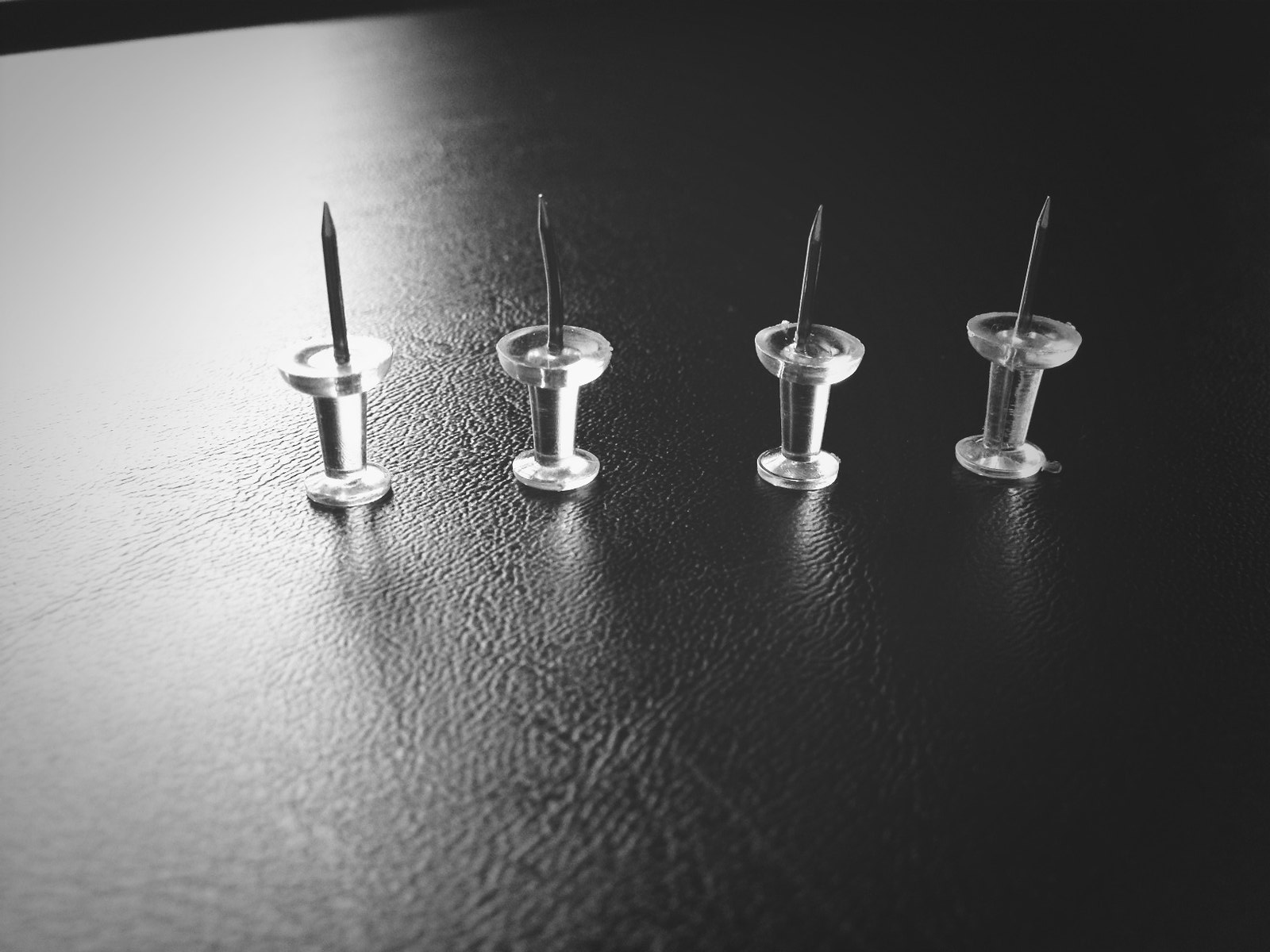The black and white photograph showcases a close-up view of four small, sharp push pins standing upright on a textured, black leather-looking surface. Each pin features a clear plastic portion and a metallic gray needle pointing upward, similar to everyday pins used for pinning items to a wall. The pins are positioned on a reflective, embossed pattern surface that contrasts both light and dark, with a strikingly lit left side and a shaded right side. One of the pins exhibits a slight bend, adding a touch of imperfection to the meticulously detailed composition. The image captures the clarity and precision of the push pins, emphasizing their minute details in a somewhat artistic, shadowy presentation.